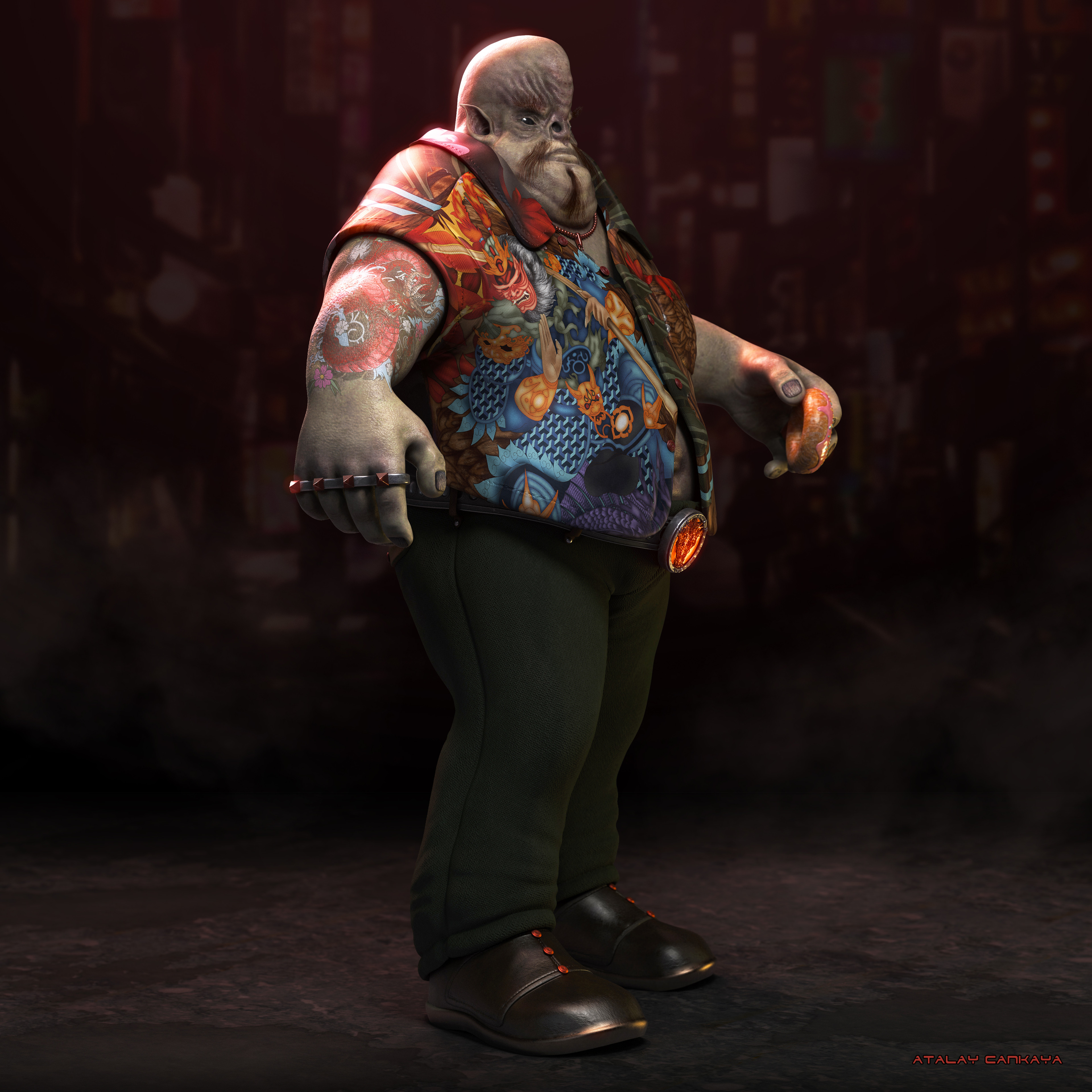The image depicts a 3D-generated humanoid alien, possibly from a movie or video game, exuding a tough, ogre-like appearance. This large character stands in a predominantly black or dark purple-gray room, partially facing the right with its muscular arms slightly spread apart as if showcasing its strength. Its gray, tattoo-covered skin features a distinctive, bald head with a protruding chin that almost connects to its chest, small black eyes, no visible nose, ears, only nostrils, and ear holes.

The alien is dressed in dark slacks or gray pants, black leather shoes with red buttons on the front, and silver soles. Its clothing includes a short-sleeved collared shirt with a vaguely Asian-inspired design: red around the upper area and sleeves, transitioning to blue towards the belly, adorned with warrior head and dragon scale motifs. It wears a belt with a bright red reflective buckle and brass knuckles on its right hand, while holding a donut in its left hand. Its left arm bears a tattoo and both hands are adorned with rings. At the bottom of the picture, the name "Atalai Kankaya" is prominently displayed in red text.